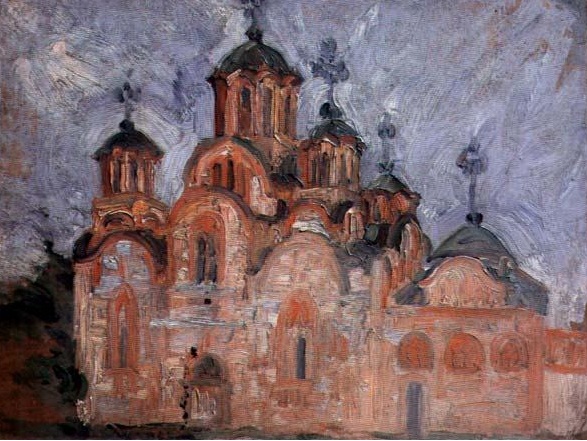This abstract painting provides a unique portrayal of a church with multiple steeples, each adorned with iron decorations. The building, constructed predominantly of stone with red stone accents around the windows and a prominent doorway at the front, stands against a textured sky painted with shades of purple, gray, and white. The tallest steeple, partly visible at the top, and several others scattered across the structure — three on the right side and one on the left — add to its striking appearance. The church itself exhibits a palette of browns, light browns, and some areas shaded with gray, while the steeples display a mix of black and gray. The ground, especially on the left side of the building, shows a blend of brown and black, with the possibility of green and brown indicating trees. The entire painting, though abstract and somewhat distorted, is richly detailed and vividly colored, presenting a clear depiction devoid of any borders, words, numbers, or human figures.